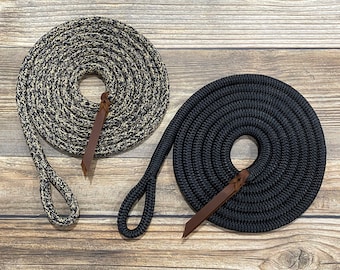The image displays two intricately coiled ropes or potential dog leashes, placed on a weathered, horizontally-planked wooden surface with a grayish and tannish hue. Each rope is meticulously woven, suggesting a high-end quality. The first rope, located in the upper left, is a marbled mix of gray and tan, forming a flat coil with a looped handle at the outer edge and a piece of brown leather trim toward the center. The second rope, positioned on the right, is solid black and similarly coiled, also featuring a looped handle on the outside and brown leather trim on the inside end. Both coils are approximately the same size, emphasizing their uniform lengths and craftsmanship.